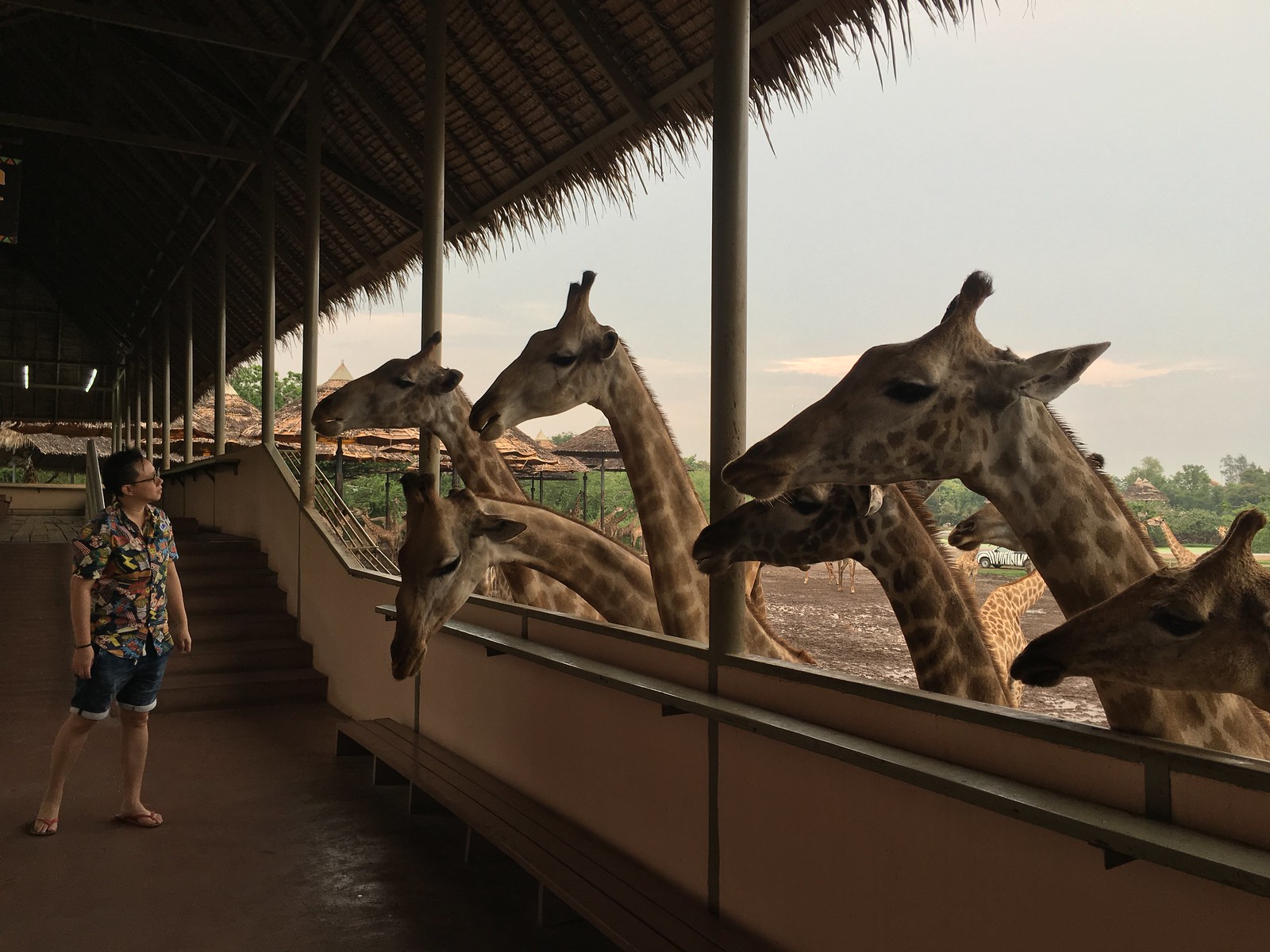In this vivid photograph, we see a young boy standing warily on a wooden walkway that overlooks a giraffe enclosure, presumably at a zoo or safari park. The boy, who sports glasses, flip-flops, dark jean-like shorts, and a colorful floral shirt, stands close to a thatched roof structure supported by wooden pillars. The roof's straw material dangles down slightly, adding to the rustic charm of the setting. Directly in front of him, seven or eight giraffes have stretched their long necks over a low wall, their heads within spitting distance. Some additional giraffes can be seen further back in the enclosure, which opens out onto a muddy field bordered by a row of trees. Off in the distance, a park vehicle hints at the presence of zoo staff. A staircase behind the boy leads up to another level of the balcony, creating an inviting yet cautious atmosphere as the boy and giraffes seem to engage in a tentative interaction.